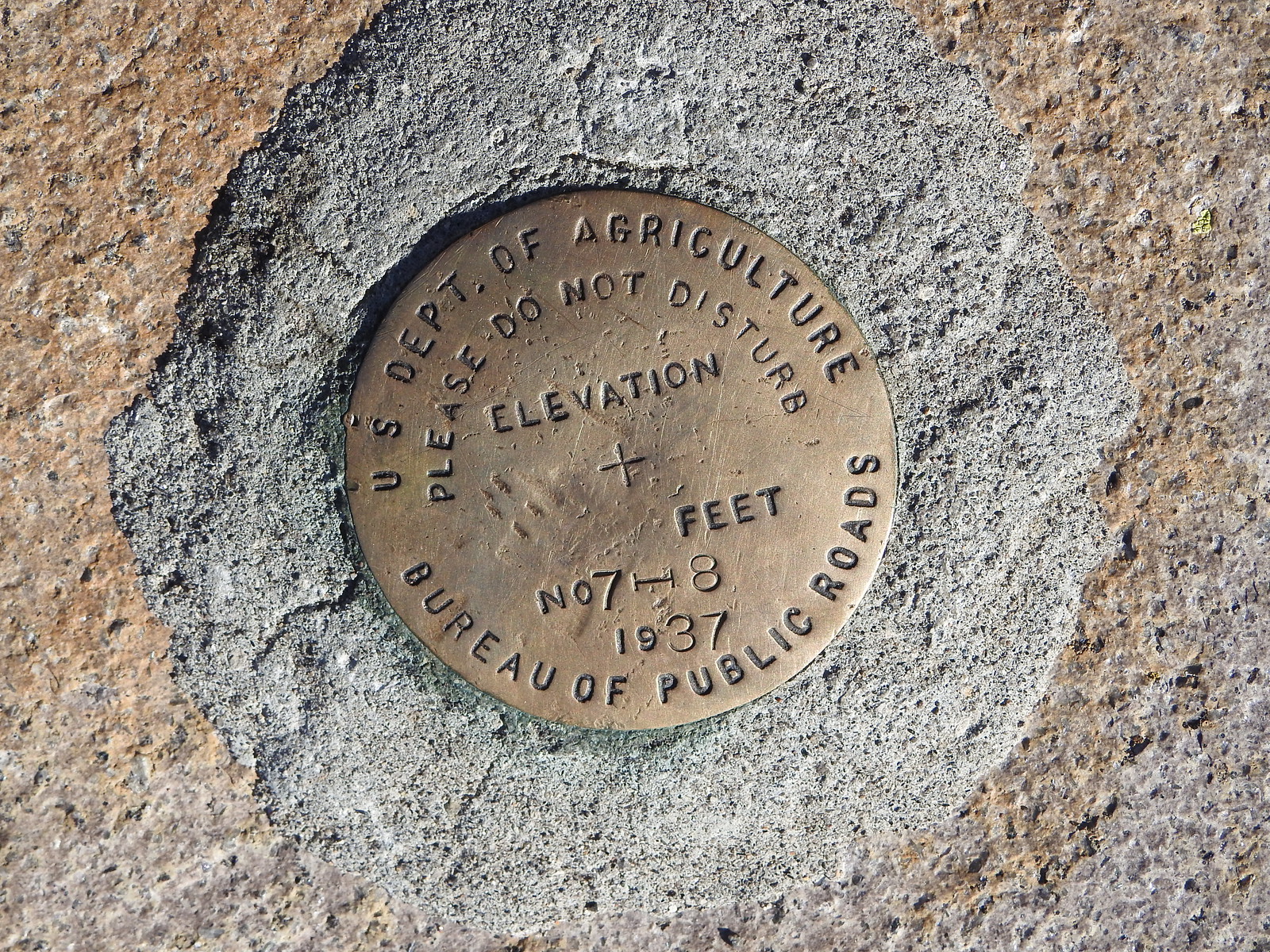Embedded within a background of light brownish and gray concrete, the image features a centrally located gold or goldish-bronze circular medallion. This medallion contains black uppercase stamped lettering. At the top curve of the medallion, it reads "U.S. Department of Agriculture" followed by "Please do not disturb." In the center, the word "ELEVATION" appears above a plus sign (+), with the word "FEET" adjacent to it. Below this, there’s a sequence that reads "N078" and the date "1937." At the very bottom arc, it states "Bureau of Public Roads." The plaque, likely an elevation marker, is set in the middle of a square photograph, surrounded by the textured gray and brown stone or cement background.